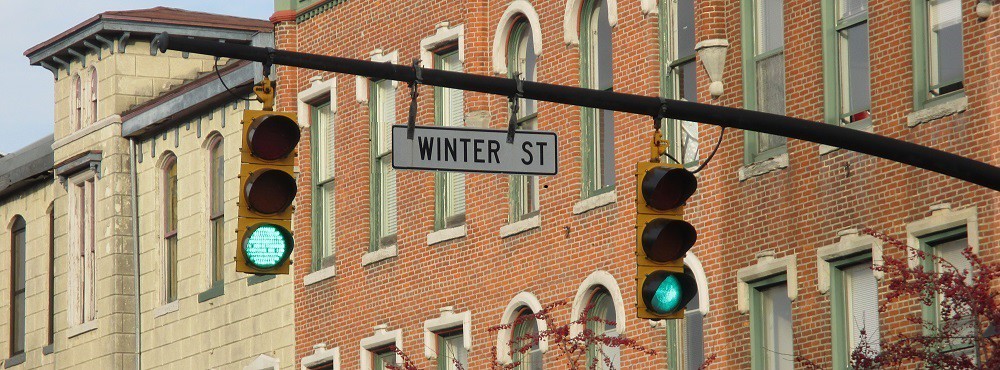This image captures an outdoor urban scene featuring two prominent streetlights, one positioned on the left and the other on the right, both emitting a green light. Centrally located between the streetlights is a rectangular street sign with a white background and black text, reading "Winter S.T." In the background, two distinct buildings are visible. The building on the right is constructed with red bricks, while the building on the left has a tan-colored facade. The architectural details of the buildings add depth and character to the picturesque street view.